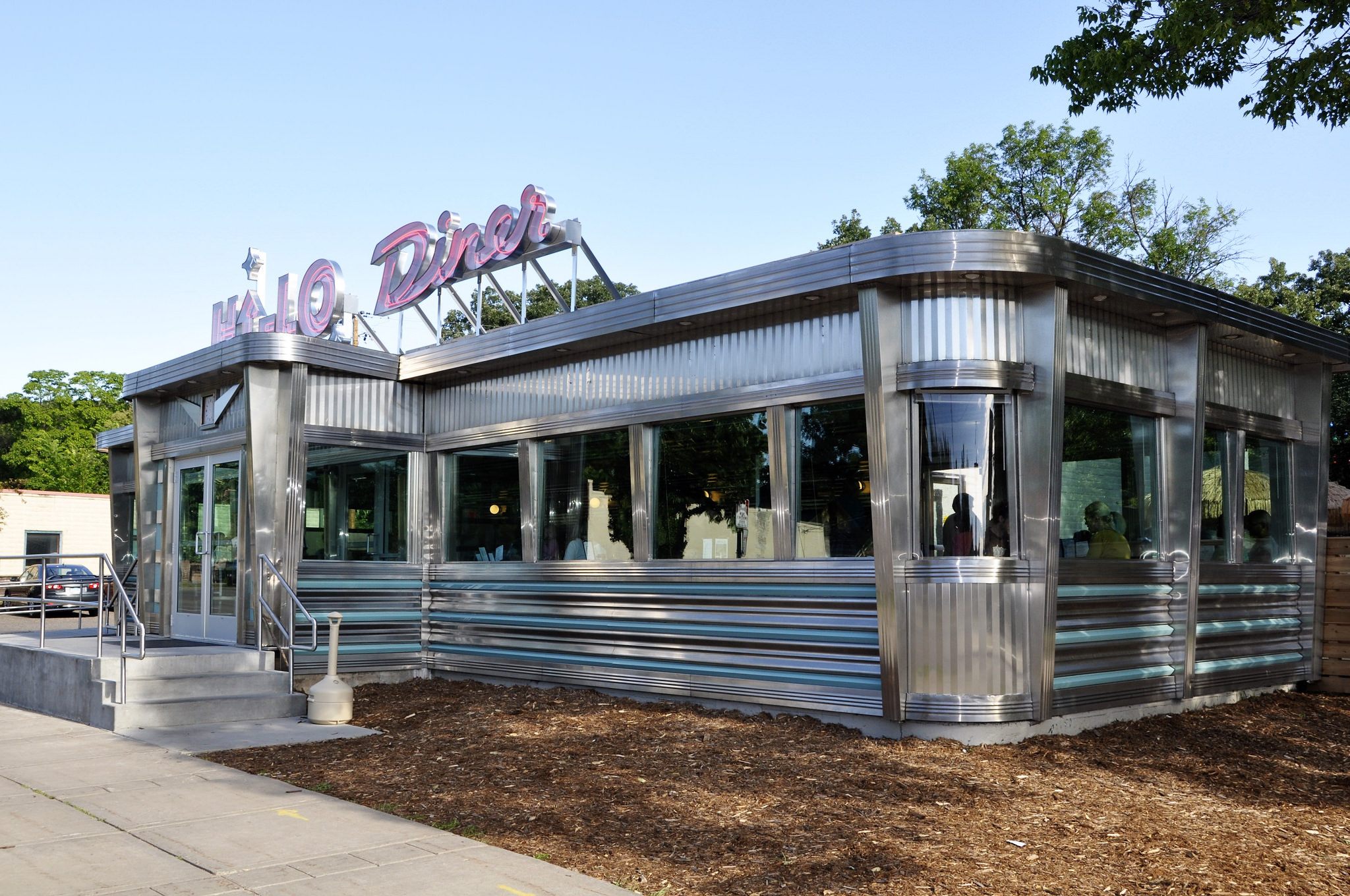This image captures a retro-styled American diner, named "Mellow Diner," designed to evoke the 1950s aesthetic. The entire exterior is constructed from shiny, reflective stainless steel, with the corrugated texture adding to its nostalgic appeal. A prominent neon sign displaying "Mellow Diner" sits atop the roof. The building features rounded corners and large windows that are separated by vertical strips of metal, perfect for offering inside views of patrons seated in booths. Below the windows, there are bluish-gray stripes running horizontally across the metal facade. A double glass door serves as the main entrance, accessible by a few concrete steps with a railing, and accompanied by a cigarette disposal container. The diner is surrounded by bark dust and has a concrete sidewalk on the left, with deciduous trees in bloom around it. The presence of a modern car in the background indicates that this diner, while nostalgically designed, exists in a more contemporary setting, making it a standout visual landmark and a clever marketing gimmick.